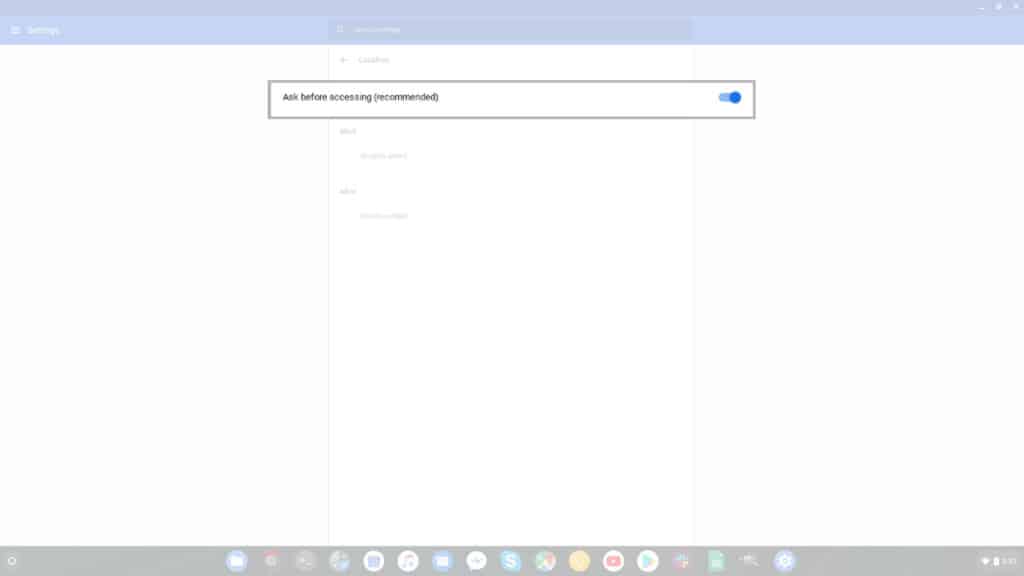The image is a screenshot, presenting a rectangular view of a desktop interface. Dominating the top of the image is a blue menu bar, characteristic of a typical desktop screen. The leftmost section of this bar contains what appears to be two or three lines, potentially indicating a settings menu. Centrally located within the menu bar is a gray, rectangular search box, occupying roughly one-third of its width.

Directly beneath this menu bar, a dropdown menu is faintly visible, suggesting that a button has been clicked to reveal additional options. Within this dropdown, subtle text is legible, consisting of about three or four words.

The most discernible element in the image is a box containing the text "Ask before accessing (recommended)." Adjacent to this phrase, a blue toggle switch is visible, indicating an active setting.

At the bottom of the screenshot, the darkened taskbar displays various icons, including those resembling iTunes and YouTube, among others. However, the focal point of the image remains the descriptive box with the toggle switch, as the rest of the background is largely obscured or grayed out.